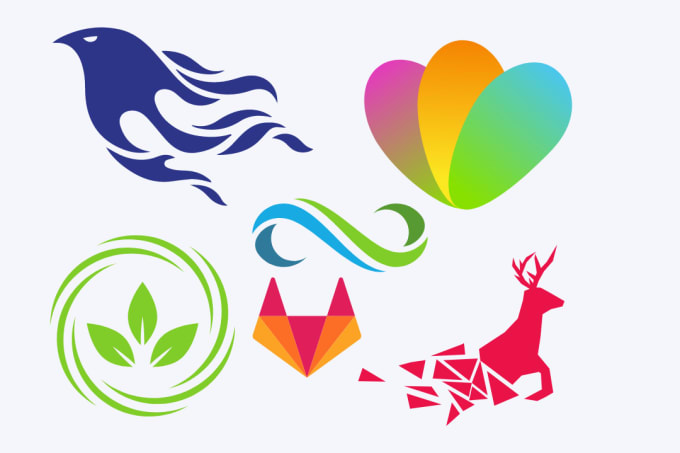The image features several simplistic shapes set against an off-white background. In the top left, a dark blue bird faces left, with its body and wings composed of wave-like designs. Below it, three green leaves are encased in a green circle formed by archways. Slightly to the right, a fox-like face is illustrated using a mosaic of pink, orange, and yellow triangles, with no distinct eyes. In the bottom right corner, a deer faces right, with its back half disintegrating into pink triangles. Lastly, above the deer, there are three distinct ovals in hues of pink, orange, and green. All shapes appear to be stylistically artist-rendered or computer-generated.